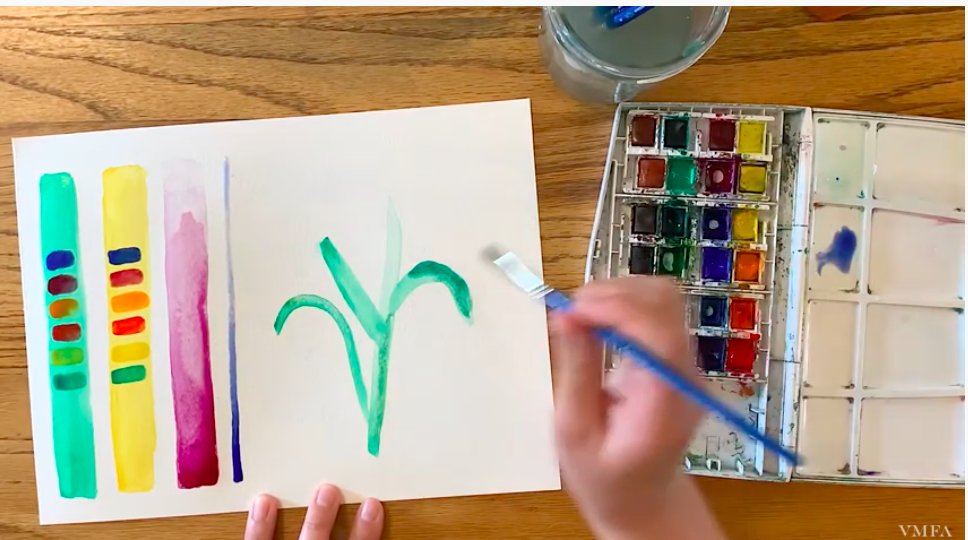The photograph captures the hands of a child in the midst of a painting activity, viewed from above, giving the perspective of the child looking down at their work. The setting is a brown wooden desk with a white piece of paper at its center. The paper displays the beginnings of a colorful creation; on the left, there are three vertical stripes—green, yellow, and pinkish-red—each with various colors swiped across, except for the pinkish-red stripe which remains plain. A dividing line separates these stripes from the rest of the paper. To the right side of the paper, the child is meticulously drawing what seems to be the stem and leaves of a flower using green paint. The child's right hand, blurred and in motion, grips a paintbrush while the left hand holds the paper steady at its edge. The paintbrush notably has a blue handle. On the desk to the right of the paper, there's a well-used watercolor paint tray housing an array of colors including blue, orange, yellow, green, brown, and black. Above the scene, a white booklet lies partially obscured by a glass filled with murky paint water, indicating the brush has been rinsed there multiple times.